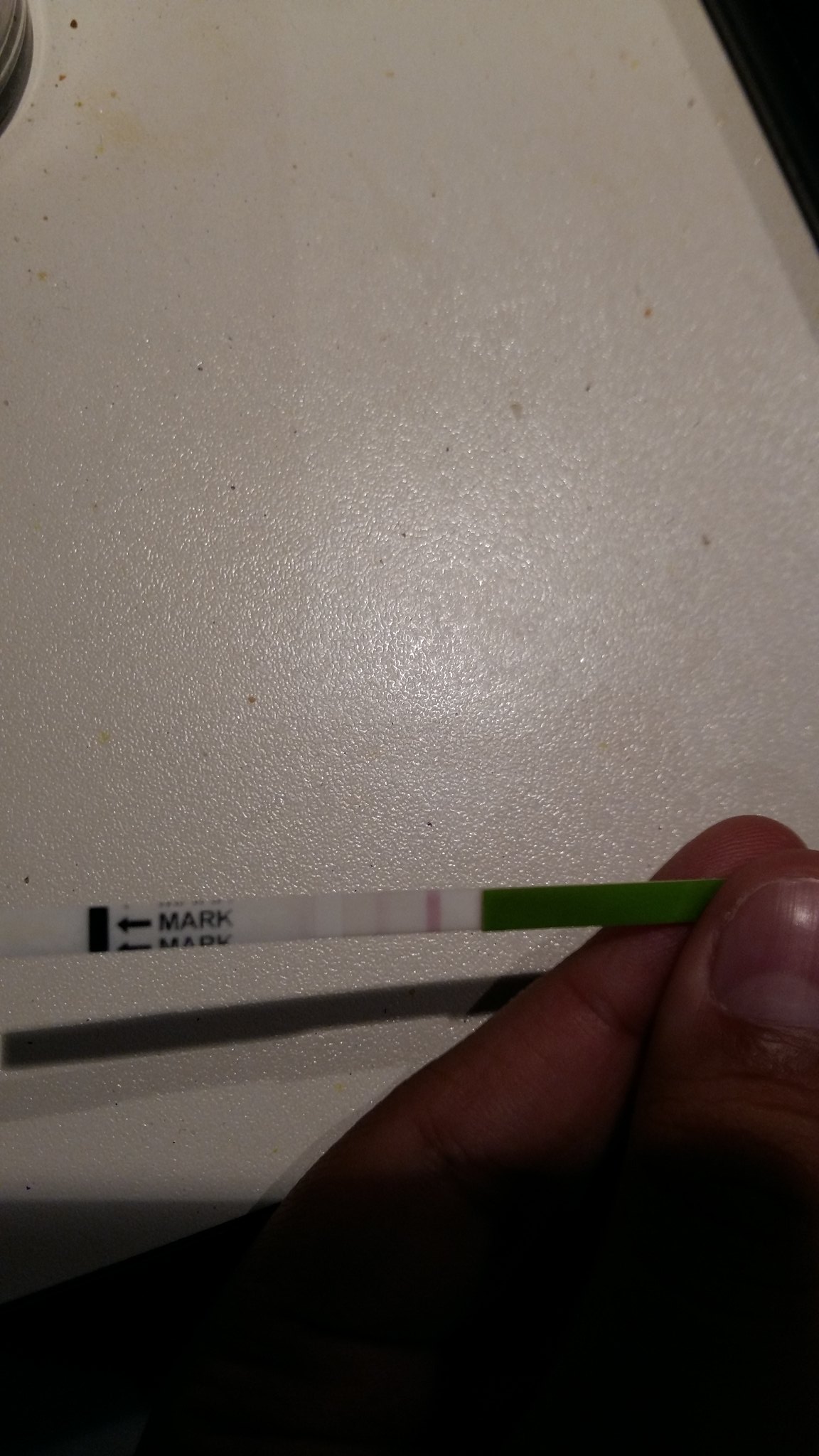The image depicts a cluttered and grimy counter surface, speckled with numerous grease spots and crumbs. Near the edge of the counter, a partially visible silver can and a black object, possibly a wall, frame the scene. In the bottom right-hand corner of the image, a left hand, of which only the thumb and index finger are partially visible, holds a testing strip. The strip displays a prominent red line and three fainter red lines against a white background. The text “M-A-R-K” appears twice, accompanied by left-pointing arrows. The strip also features a black line and a green section. Below the strip, dark and light shadows are reflected on the counter's surface. The hand casting the shadow has a portion obscured by a black circular shade.